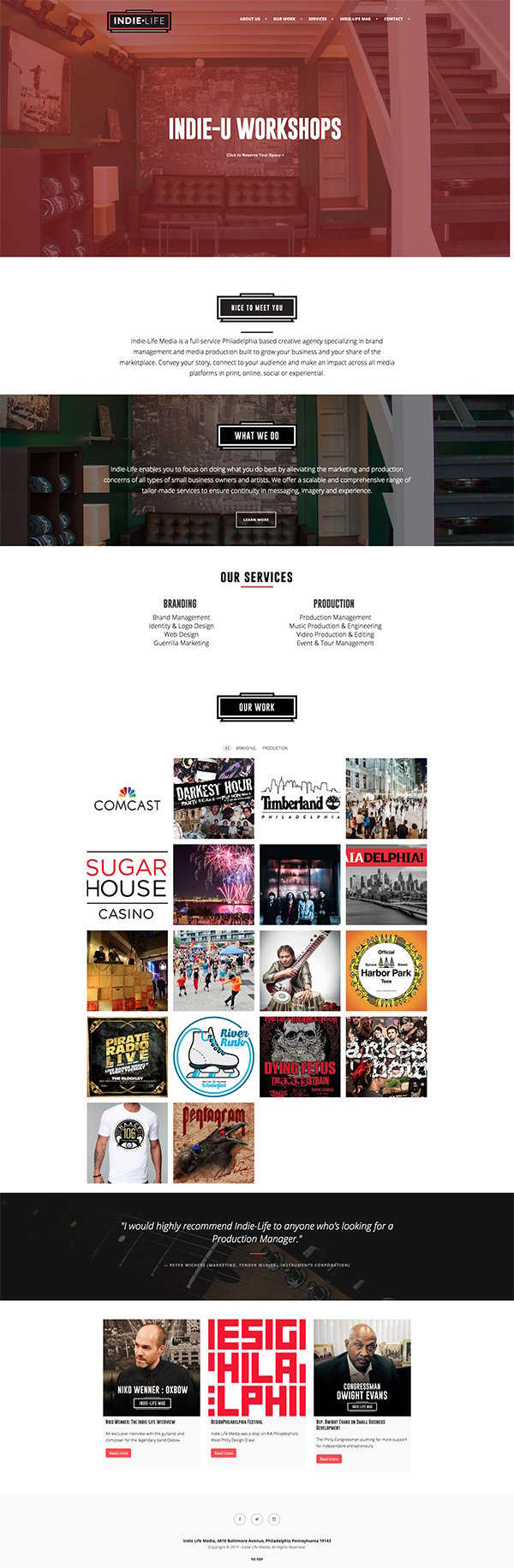The image depicts a horizontally stretched webpage of "Indie Life," with the brand name displayed prominently at the top. The navigation bar includes several drop-down options: "About Us," "Our Work," "Services," "Life," "MAG," and "Contact." Beneath the navigation bar, the largest text reads "Indie-U Workshops" in white font, centered on the page. The background features a red-tinted, cozy living room scene with visible stairs on the right. Below the "Indie-U Workshops" heading, there is a text block that reads, "Nice to Meet You. Indie Life Media is a full-service Philadelphia-based creative agency specializing in brand management and media production built to grow your business and your share of marketplace. Convey your story, connect to your audience, and make an impact across all media platforms, in print, online, social, or experiential."